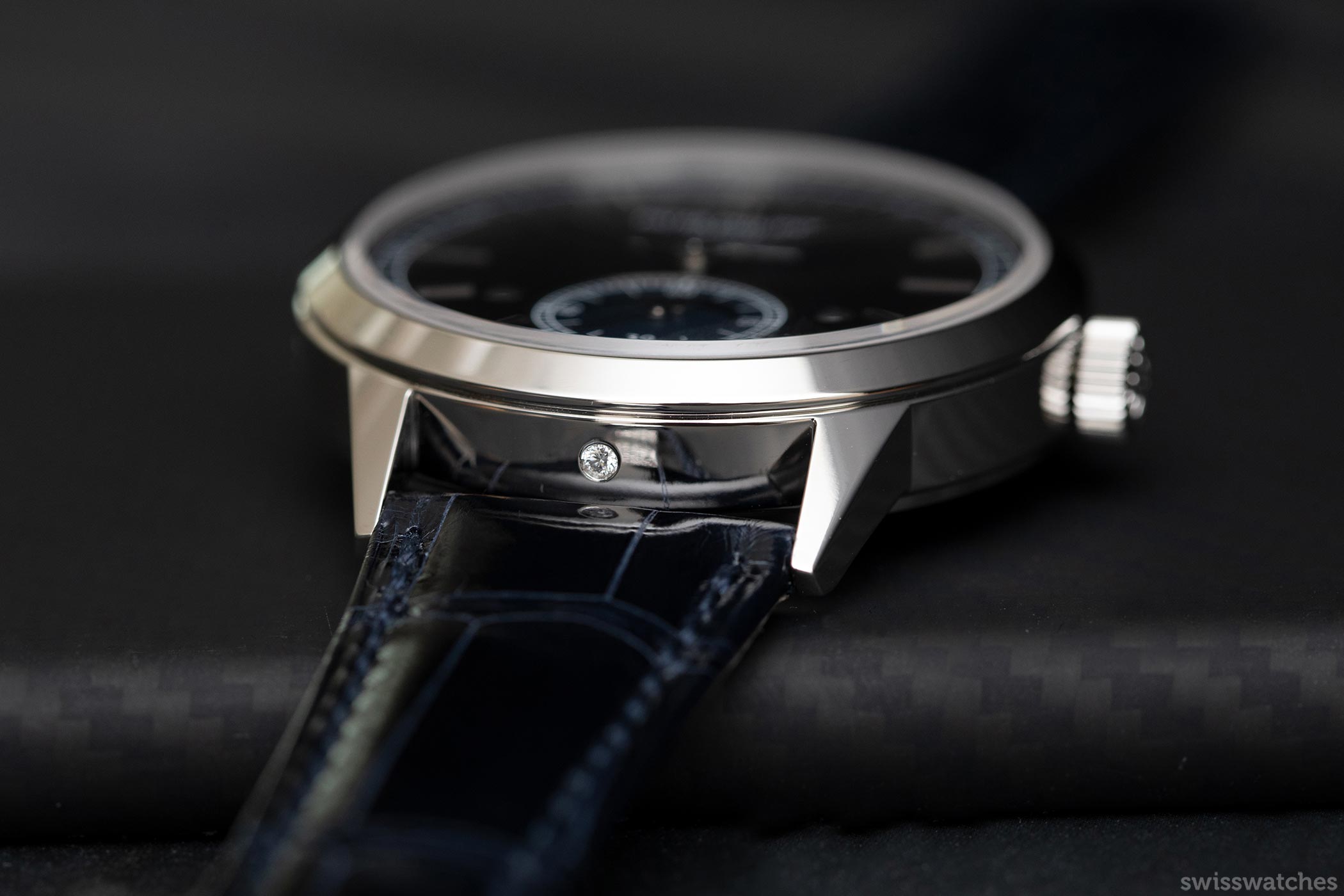This close-up horizontal image features a detailed view of a silver watch with a black face, adorned with white markings and a small knob on the right side. The watch appears to be set against a dark, velvety backdrop that enhances its sleek design. The wristbands, displaying a crocodile skin texture, have distinct white stitching and blue threads along the seams, creating a sophisticated contrast. The background transitions from a blurry gray at the top to a clearer view at the bottom, where the watch rests on a dark piece of fabric resembling a cloth or book. The text "Swiss watches" appears in light gray at the bottom right corner, adding a subtle yet elegant touch to the composition.